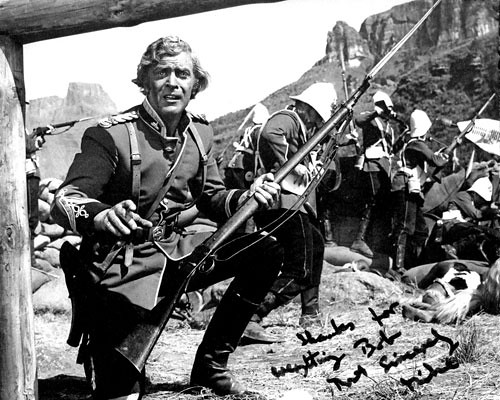The image is a black and white photograph, capturing an old and historic scene featuring a group of soldiers dressed in period uniforms, likely European from around the turn of the century. Most soldiers are equipped with long rifles, and they don white helmets, standing amidst a dry grass landscape that stretches into a background of rugged mountains and canyons visible from left to right under a pale sky. In the foreground, a man with short hair is kneeling or half-sitting, one finger of his right hand pointed while holding a rifle in his left. The ground around them is littered with bodies and bags, possibly indicating a recent battle, alongside hay that has been pushed aside and stepped on. On the top left of the image, a pole or wooden branch is visible. The photograph is signed with handwritten text in black ink on the bottom right, though the writing is illegible. The serious expression on the kneeling man's face adds to the gravity of the scene.